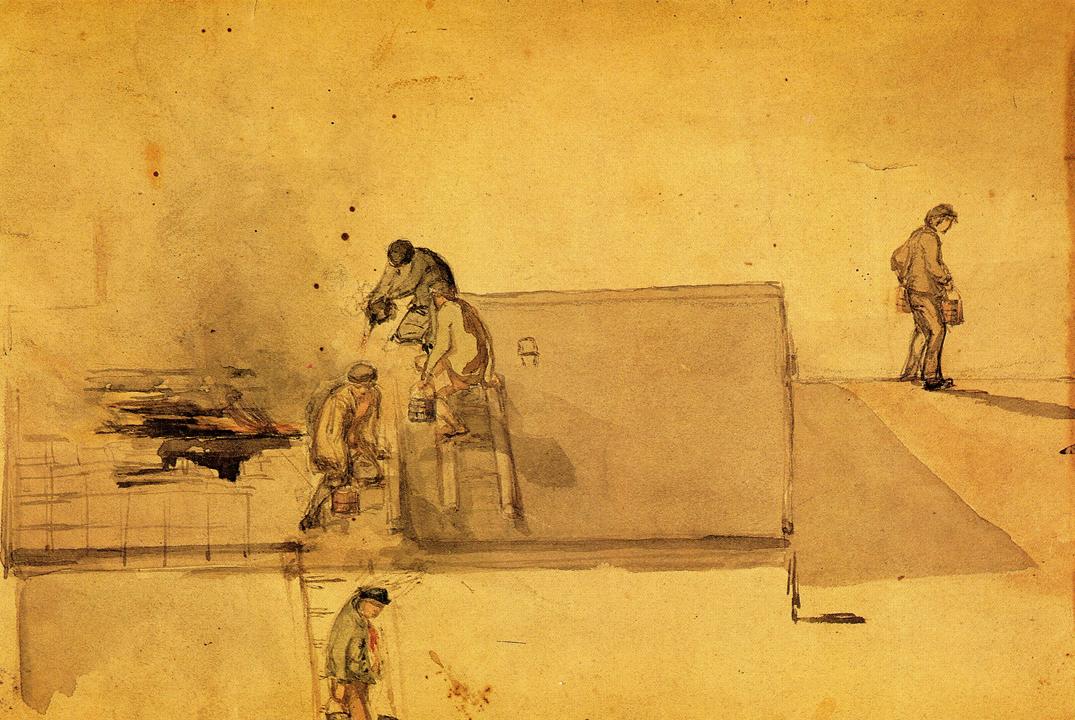This image depicts a hand-drawn painting or sketch of five men seemingly working on a building, rendered in various shades of yellow, red, orange, pink, brown, and tan, on dark yellowish, old-timey looking paper with ink blots suggesting pen, pencil, or paint usage. Central to the composition is a man standing on a three-rung ladder holding a bucket, with another man above him potentially holding a drill. The scene features several other figures: a man below the ladder handling another bucket, a person to the right also holding a bucket, and an individual walking away with yet another bucket. Some are engaged in tasks like walking or bending, possibly throwing or carrying liquid, perhaps painting the siding or working on structural elements. The setting feels industrious, reflective of construction or maintenance activities, without any visible text, amidst a yellow background that ties the various actions and objects together in a coherent artistic frame.